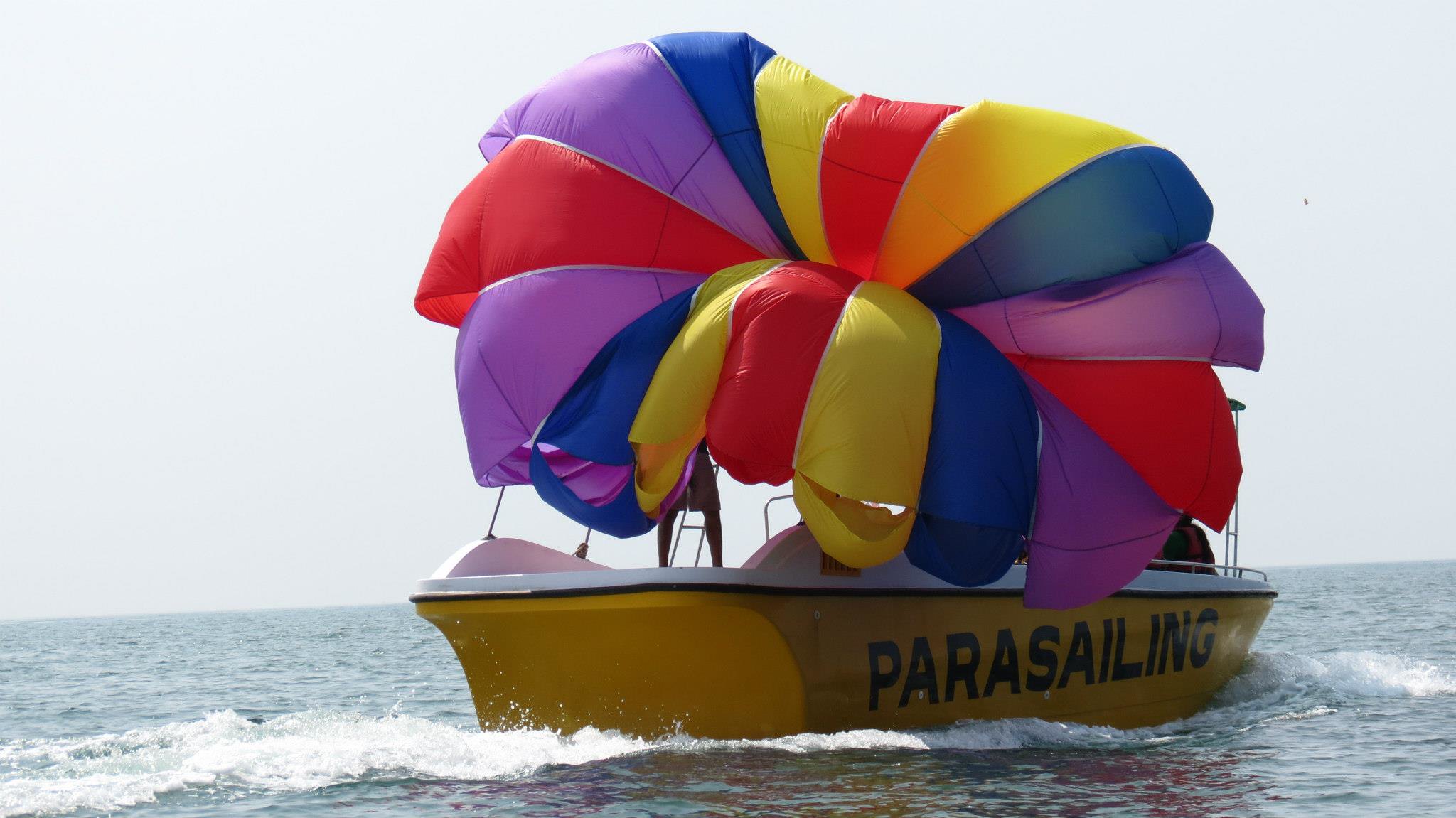Outdoor color photograph taken at daytime on the ocean in bright sunlight. The focus of the image is a power sailing boat, which is yellow on the bottom and white on the deck, with black capital lettering reading "PARASAILING" on its hull. We are viewing the boat from the back and right side, showing a three-quarter view of the stern and the right side. The boat's superstructure is largely obscured by a large, partially collapsed multicolored parachute, featuring stripes of yellow, green, purple, red, and blue, creating a slightly oval shape. The parachute, evidently used for parasailing, covers most of the boat’s deck and a person's legs are visible behind it, suggesting they are standing on the deck. The ocean water, a bluish dark green, is calm with minor ripples near the boat. The wake from the boat extends from the stern to the lower right corner of the frame, creating white splashes. In the background, the horizon blends into a pale white sky, giving a sense of open space and tranquility.